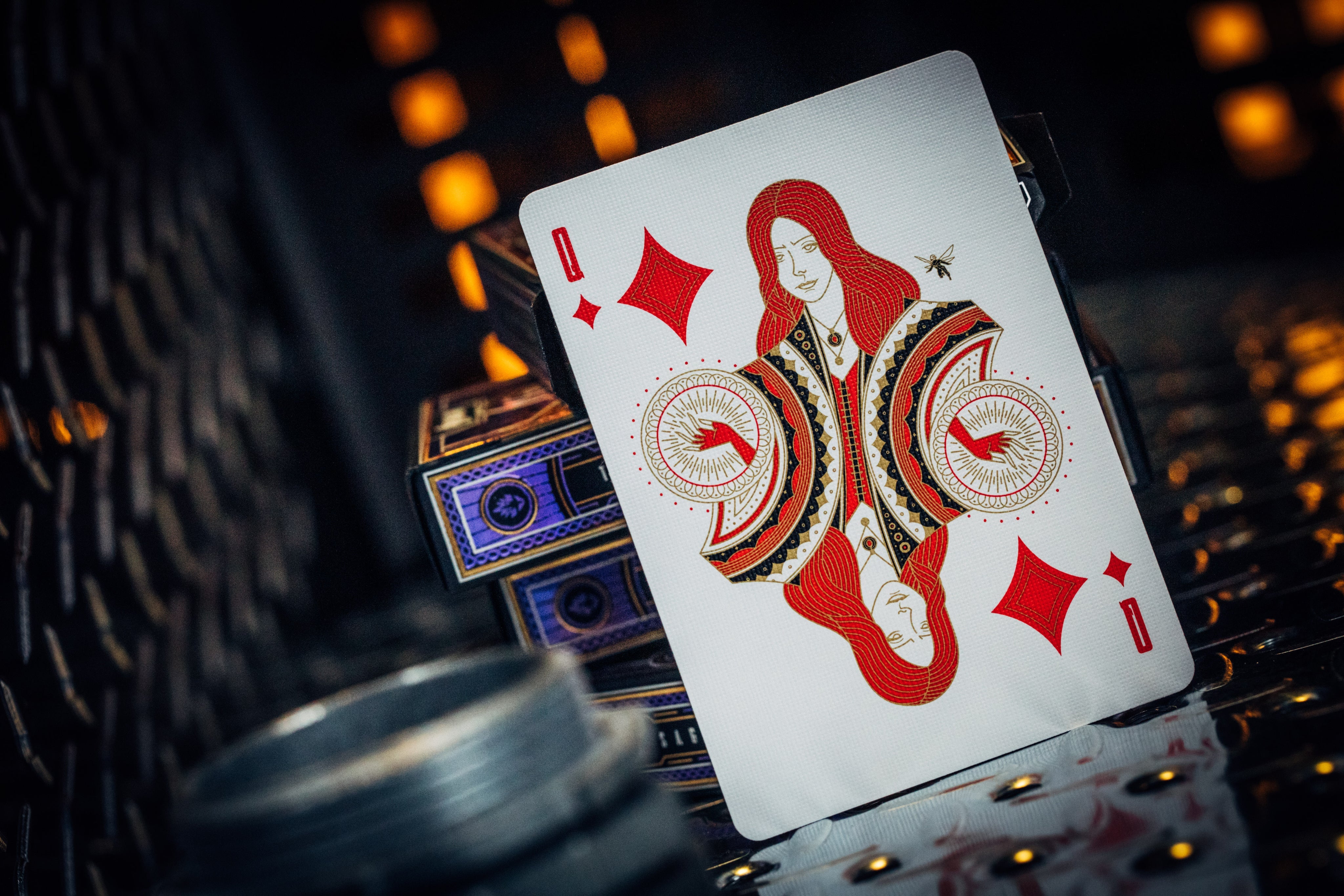This photograph captures a uniquely stylized Queen of Diamonds playing card, distinct from those found in standard decks commonly available at convenience stores or casinos. The card's artwork features a character with flowing, very long red hair, striking a pose that suggests she possesses magical powers, reminiscent of the Scarlet Witch from the Marvel movies. The figure is depicted with what appear to be supercharged energy circles around her hands, enhancing the comic-book-like feel of the design. Interestingly, there seems to be a small, fairy-like figure, possibly akin to Tinkerbell, hovering in the dimly lit background. The card is propped up against four boxes of cards, ensuring its intriguing design is fully visible against the dark setting.